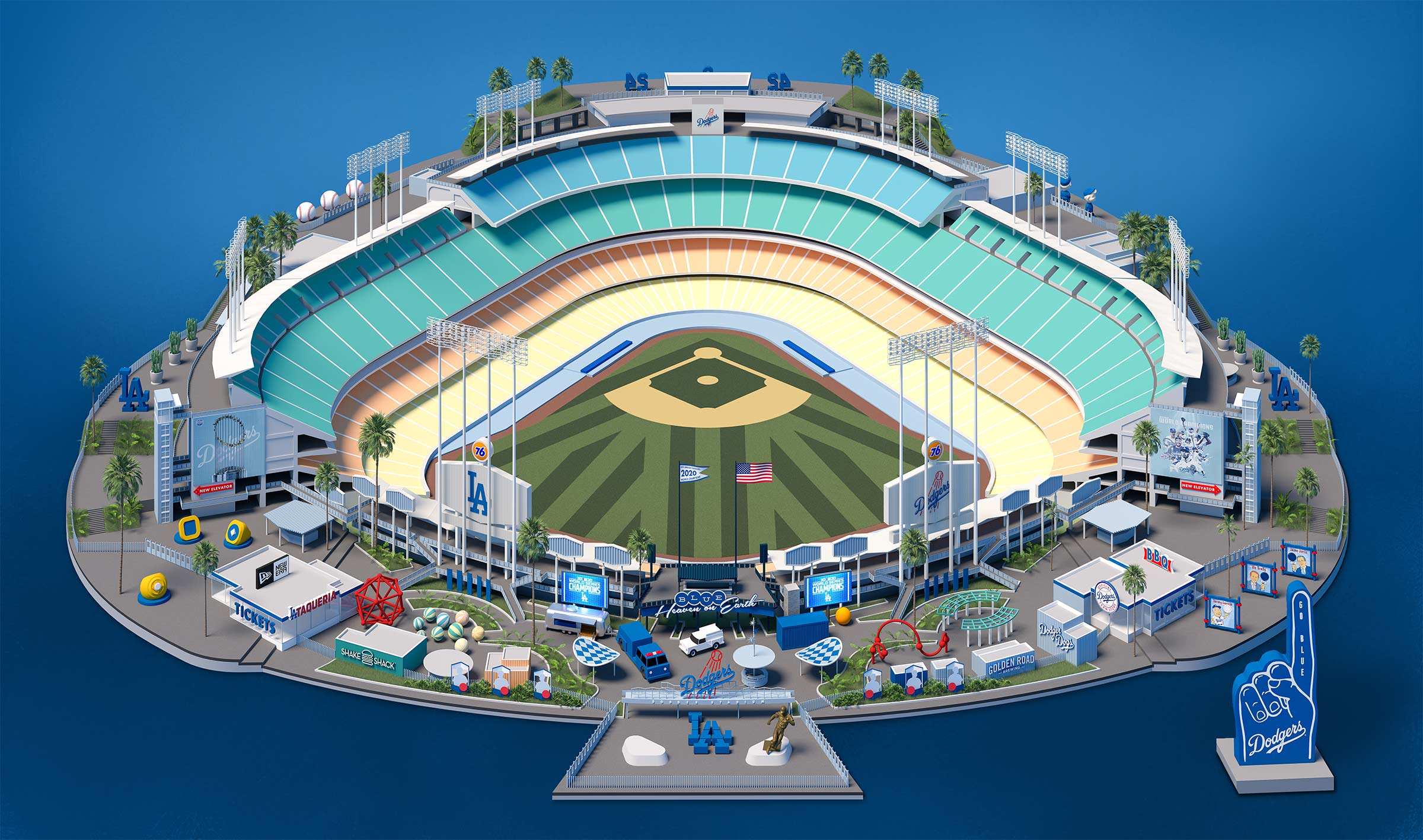The image is an animated, illustrated diagram of a stadium, possibly from a game or a stadium design concept. The stadium, diamond-shaped and centrally located, is depicted from an aerial perspective. The background transitions from a lighter shade of blue at the top to a darker shade of blue at the bottom, suggesting depth or sky.

Surrounding the stadium are various small buildings and shops, such as "Tickets," "Shake Shack," and "New Era," positioned towards the front. The text inscriptions also include "LA Dodgers," "Blue heaven on earth," "Champions," "L.A. Tequira," "New elevator," "76 L.A.," and "2020."

The major colors featured are blue, aqua, turquoise, yellow, beige, green, dark green, black, gray, red, and white. The stadium includes a pitch area, stands for spectators, and surrounding roads and car parks for utilities.